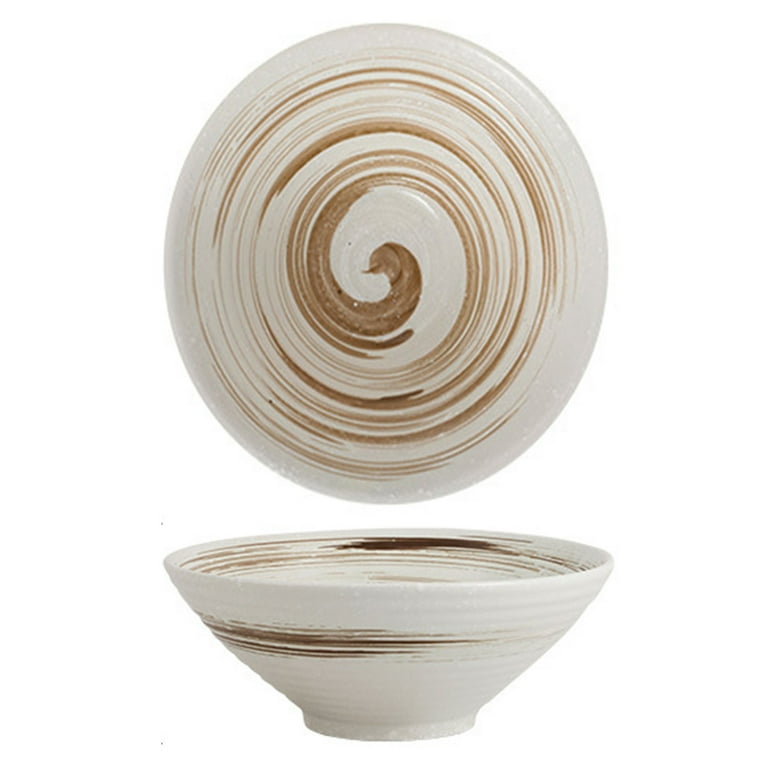This image showcases a pair of ceramic items on a stark white background, emphasizing their detailed craftsmanship. The composition features an off-white plate adorned with intricate brown swirls, positioned at the bottom. Above it, centrally aligned, is an off-white bowl depicted from two perspectives: a side view and a direct aerial shot. The bowl, larger than the plate, displays matching brown swirls both inside and out, spiraling to its base. The ceramics appear smooth and pristine, hinting at their newness. Their thick construction suggests durability, with slight imperfections like bubble-induced holes adding rustic authenticity. The lack of additional colors or text highlights the simplicity and elegance of the pottery's design, making the brown and white hues stand out vividly against the clean background.